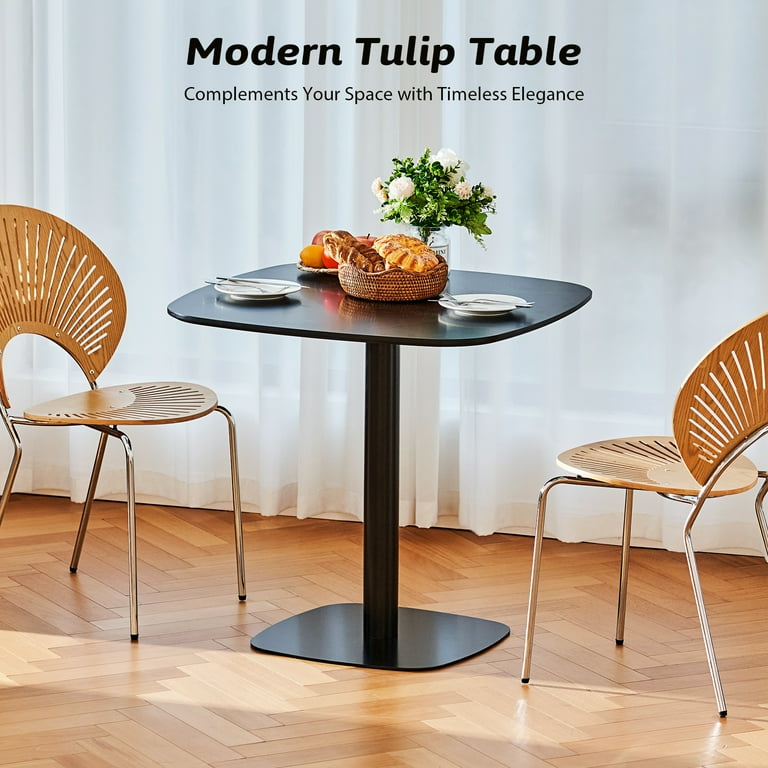In this photograph, which appears to be an advertisement for furniture, we see a small black table with two wooden chairs, each featuring a circular seat and a backrest with horizontal notches, supported by metal legs. The table is adorned with two white plates, each set with a fork and knife, and a small basket containing freshly baked bread at its center. A glass jar filled with white flowers and green leaves is placed adjacent to the basket. Behind this arrangement, a sheer, flowing white curtain partially covers a large window or door, allowing light to softly illuminate the scene. The floor consists of light wooden rectangular planks, adding to the room's warm and inviting ambiance. The top of the image features black text that reads "Modern Tulip Table," with a subheading in smaller black text, "Complements your space with timeless elegance.”